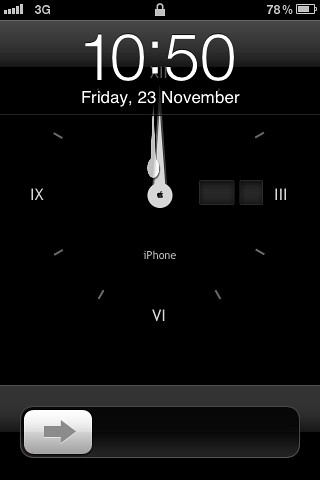This is a detailed screenshot of a lock screen on an iPhone, showing various elements of the device's interface. The iPhone displays full signal strength with five bars and is connected via 3G, as indicated by the status bar at the top. The battery level is at 78%. The digital clock on the screen reads 10:50 AM, Friday, 23 November. The lock screen features an analog clock positioned prominently in the center, adorned with Roman numerals, and labeled "iPhone" underneath. The analog clock indicates a different time with its white hour and minute hands both pointing upward. Additionally, there are two small sections displaying the day and date. At the bottom of the screen, there is a slide-to-unlock banner with a small gray arrow pointing to the right.